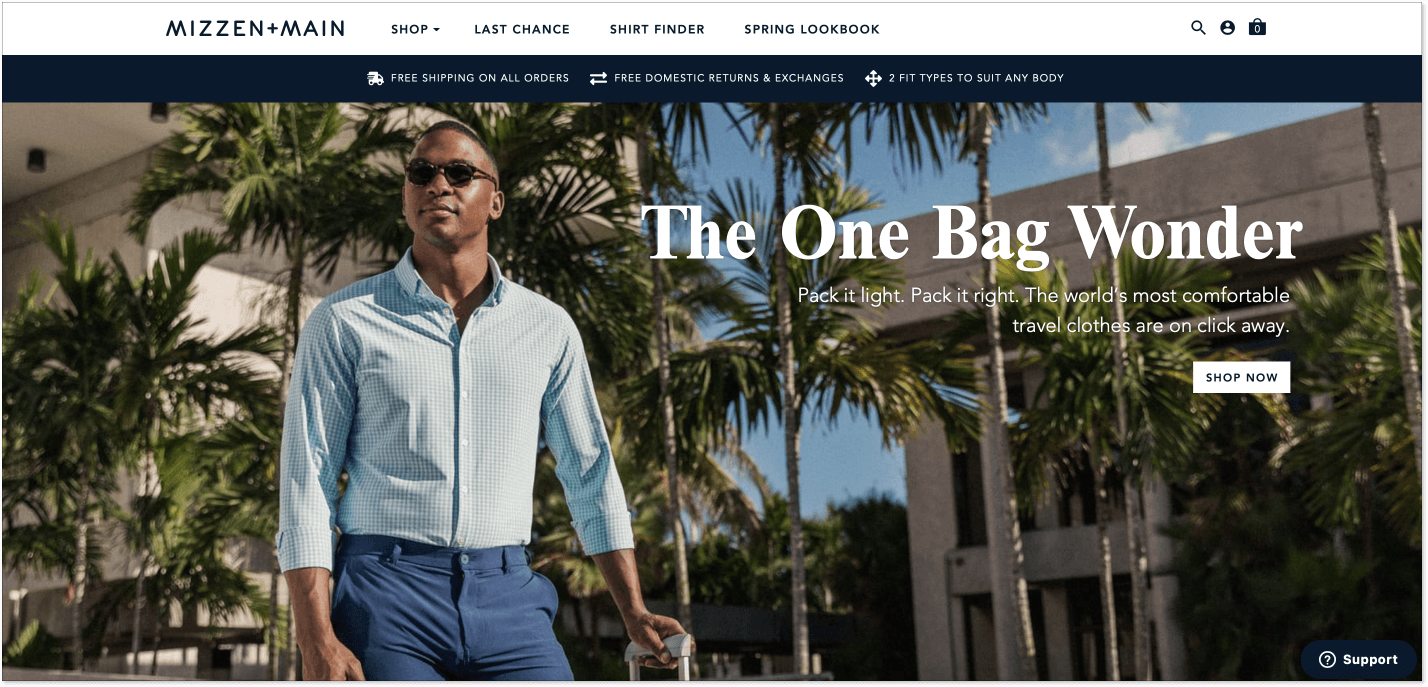The webpage features a stylishly dressed African American man, wearing sunglasses, a blue shirt, and blue pants. He appears to be holding the handle of a piece of luggage. The background showcases multiple buildings and trees, including several palm trees, indicating a daytime setting under a clear blue sky. At the top of the page, the text "Mizzy Man" is prominently displayed. The navigation menu includes options such as "Shop," "Last Chance," and other related categories, suggesting that this webpage is for an online shopping platform. Additionally, there's a support button located at the bottom right and a "Shop Now" button, emphasizing the shopping functionality of the site. The man in the image is gazing off to the corner, adding a sense of depth and thoughtfulness to the scene. Overall, the webpage is well-designed and visually appealing, without any noticeable issues.